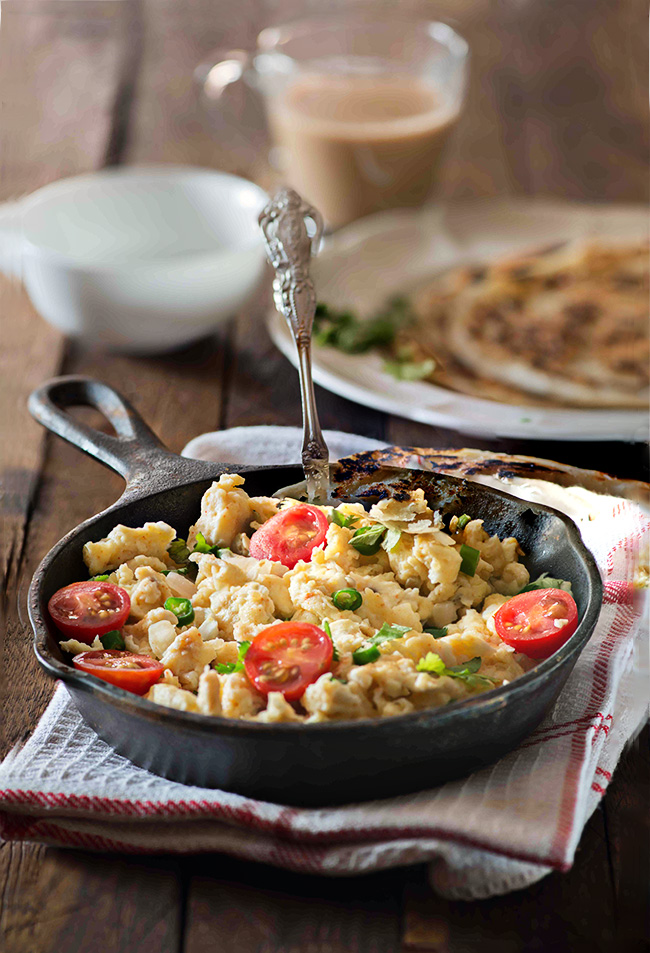A beautifully curated photograph showcases a delightful scrambled egg dish served in a black cast iron skillet, positioned just below the center of the image. The dish is garnished with finely sliced green onions, parsley, and five halved cherry tomatoes, adding vibrant colors to the presentation. The cast iron pan, bearing visible burn marks that hint at its cooking history, rests on a red and white kitchen towel. A spoon with a silver handle protrudes from the pan’s edge, ready for serving. The skillet’s handle extends to the left, anchoring the composition on what appears to be a brown wooden table. In the background, a white plate with what looks like pancakes and a glass cup of brown liquid, likely tea or coffee, along with a small white bowl, complement the rustic and homely setting. This image, with its meticulous attention to detail, exudes the charm of a food blog post, inviting viewers to savor the tempting culinary creation.